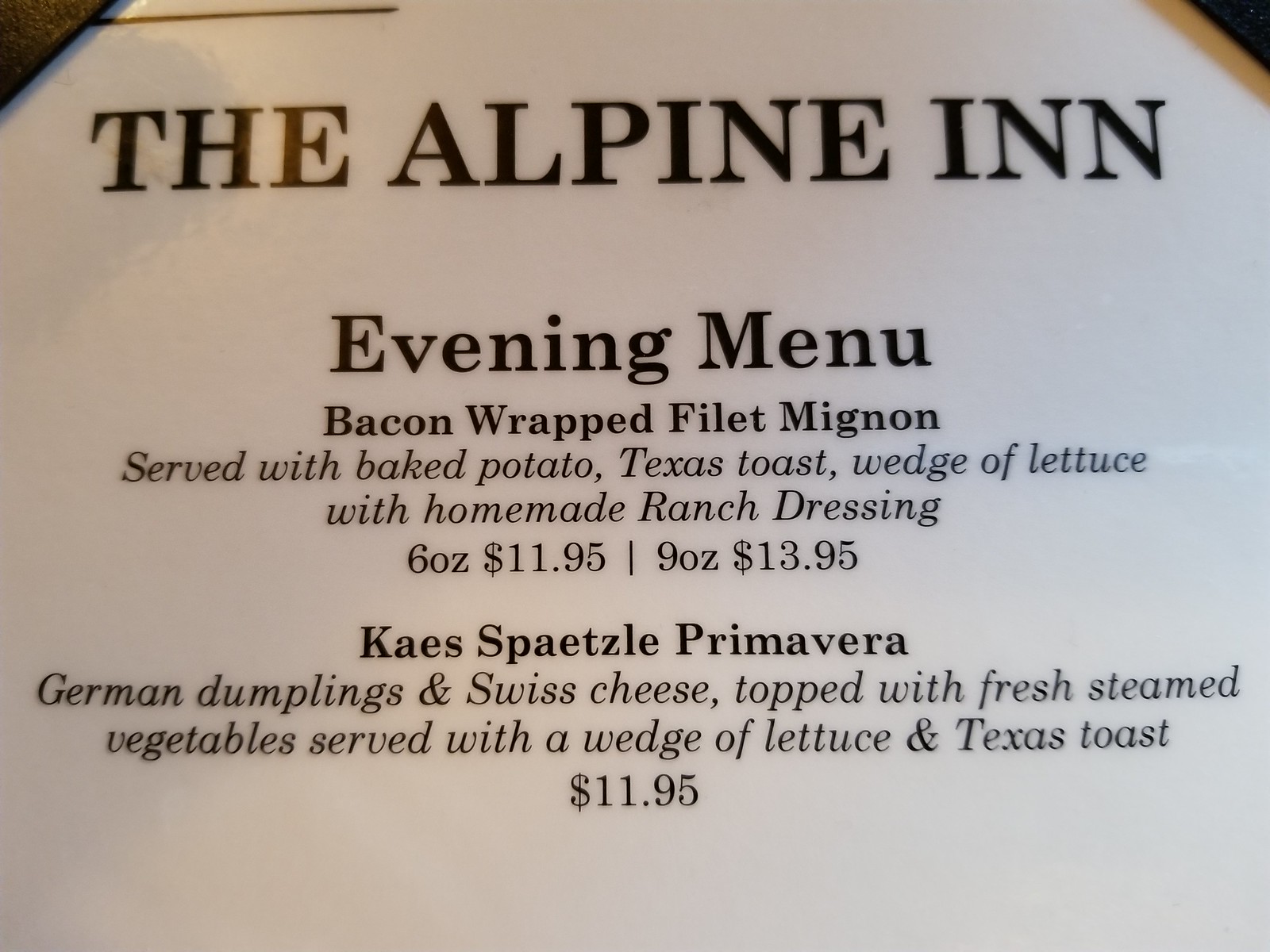This image features a close-up view of the upper section of a restaurant menu. The menu is framed by small pleather tabs at both the upper left and right corners, which secure it in place. A touch of gold trim is visible near the top edge, adding a hint of elegance. The menu itself consists of black type against a clean white background. At the top, bold capital letters read "The Alpine Inn," indicating the name of the establishment. 

Below this title, the heading "Evening Menu" introduces the dining options. The first listed entrée is a bacon-wrapped filet mignon, served with a baked potato, Texas toast, and a wedge of lettuce with homemade ranch dressing. This entrée is available in two sizes: a 6-ounce filet priced at $11.95 and a 9-ounce filet for $13.95.

The second option is "Spätzle Primavera," which features German dumplings and Swiss cheese topped with freshly steamed vegetables. This dish is also served with a wedge of lettuce and Texas toast and is priced at $11.95.

The image captures only this top portion of the menu, leaving the viewer to assume there are additional selections on the unseen parts.